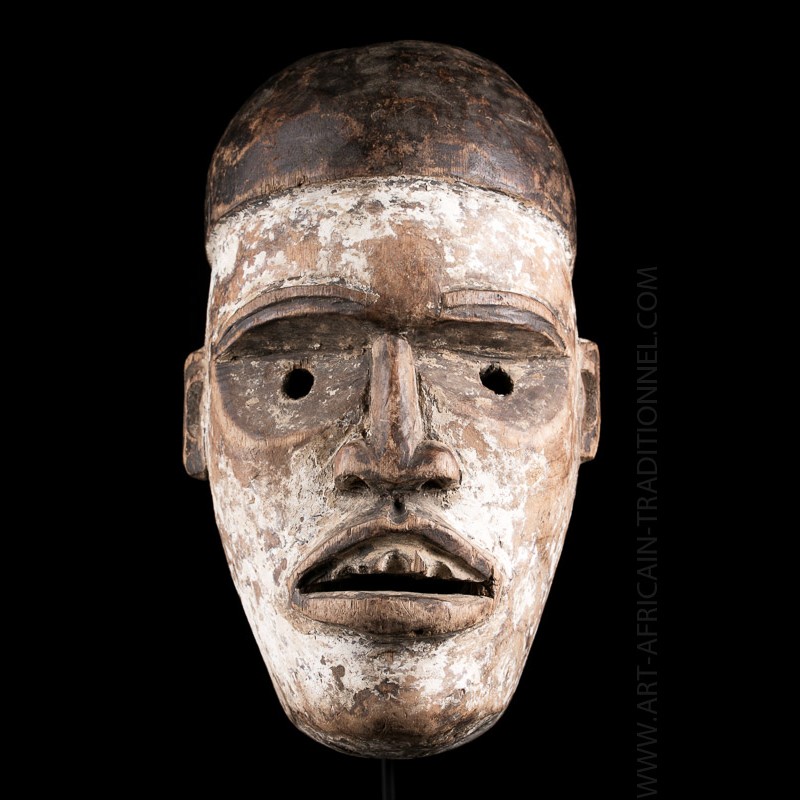This photograph showcases a traditional African tribal mask carved from wood, set against a solid black background. The website watermark, www.art-african-traditional.com, runs vertically along the right side of the image. The mask features a distinct, elongated face with a broad, manly chin. Its top is a dark brown dome, while the face itself is a lighter brown, whitewashed in places, giving the wood a distressed, aged appearance. Intricately carved eyebrows and eye sockets are highlighted, with actual holes cut out for vision, suggesting the mask was designed to be worn. The slightly parted mouth reveals upper teeth that are accented with white pigment, adding to the mask's eerie and ancient look. Carved ears on either side of the mask complete the facial features, presenting a vivid representation of traditional African craftsmanship.